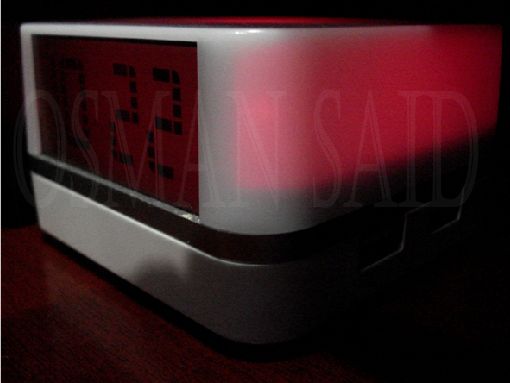The photograph captures an alarm-style clock or possibly a clock radio, set in a dimly lit environment. The clock, which appears to have a rounded square shape though it might be triangular, is shrouded in heavy shadows, revealing only two of its faces. The camera angle presents a view from one of its rounded edges. The LED display diagonal to the lens shows the time as 22 minutes past an unspecified hour, with the visible numbers situated at the clock's right side. The display extends towards the back left of the image. A striking red highlight, likely from a nearby light source, streaks horizontally across the clock's upper right surface, contrasting starkly against the deep shadow engulfing the lower portion, where the clock descends into complete darkness.